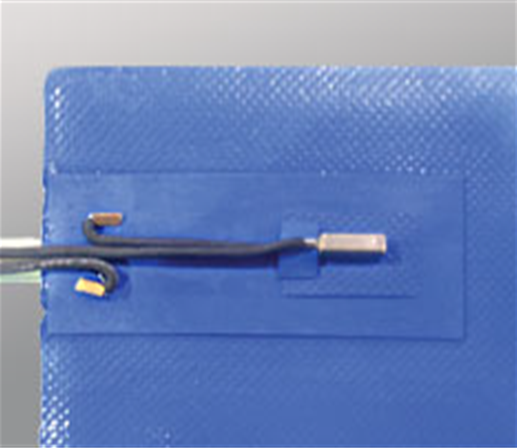This photograph showcases a close-up of a blue, square-shaped lid with a metal handle, set against a light gray, silver-toned background. The lid appears to be made of a shiny, textured material, possibly vinyl, designed with a diamond pattern that suggests it is a protective cover, perhaps akin to an iPad case. The image captures the top left corner of the lid while the other sides are cut off, obscuring the contents beneath. A notable feature is a set of three black wires extending from a metallic silver connection point on the blue lid. These wires fan outwards, with two ending in distinctive, curved metal tips; one is orange, curved back toward the product, while the other is yellow, curved outward. The item appears to be some form of electronic device, although its specific use remains unidentified.